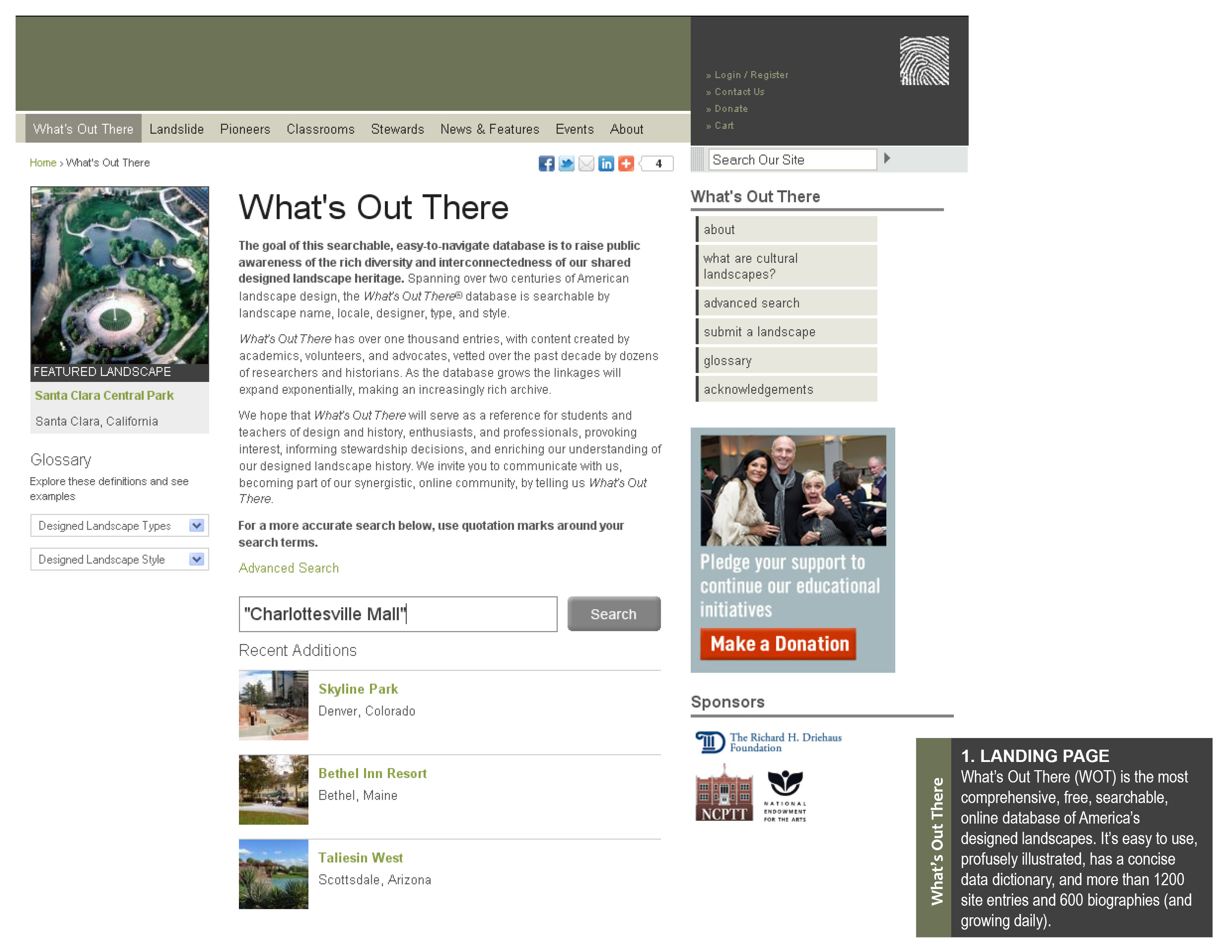The image captures a website layout focused on landscape design heritage. At the top of the webpage is a blank olive green banner, followed by a khaki-colored menu bar. The initial menu option, titled "What's Out There," features a gray background with khaki-colored text. The menu lists the following options in black print: Landslide, Pioneers, Classrooms, Stewards, News and Features, Events, and About.

On the right-hand side, from top to bottom, there is a black square containing the options: Log In/Register, Contact Us, Donate, and Cart. Above these options, a fingerprint icon is visible, with a grey background underneath. Adjacent is a white search bar labeled "Search Our Site."

Further down, the background turns white with the text: Home, What's Out There. Below this text, an image of a landscape is displayed, captioned "Feature Landscape: Santa Clara Central Park, Santa Clara, California." The accompanying description reads: 

"The goal of this searchable, easy-to-navigate database is to raise public awareness of the rich diversity and interconnectedness of our shared design landscape heritage. Spanning over two centuries of American landscape design, the 'What's Out There' database is searchable by landscape name, locale, designer type, and style."

Additional details explain more about the database, followed by an advanced search option. Below this, the text reads "Recent Additions," including entries such as Charlottesville Mall, Skyline Park, Bethel Inn Resort, and Tavis Inn West in Scottsdale, Arizona.